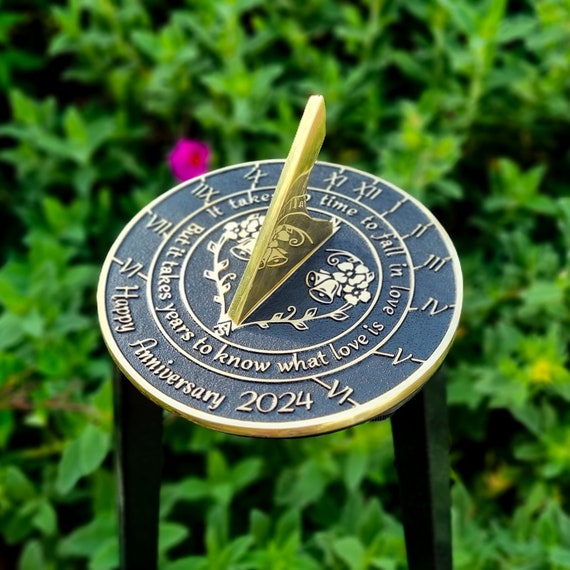The image captures a meticulously crafted sundial, prominently featured at the center of the photograph. This outdoor shot, taken during the daytime, showcases the sundial mounted on three sturdy black legs. The sundial itself is slate gray with intricate gold embellishments highlighting various elements. Surrounding the central dial, gold rings encircle Roman numerals from I to XII, directing attention towards the reflective, gold-colored gnomon, which casts the shadow to indicate time.

In the heart of the sundial, a decorative centerpiece features a heart shape adorned with vines, flanked by flowers and bells on either side. The captivating inscription reads, "It takes time to fall in love, but it takes years to know what love is," thoughtfully encircling the centerpiece. Below this profound message, in bold, golden lettering, the sundial commemorates a special occasion with "Happy Anniversary 2024."

The background of the image is slightly out of focus, emphasizing the sundial's details. Behind it, there's a delightful yet blurry mix of green plants and a singular pinkish-red flower, offering a subtle contrast to the sundial's sharp, clear features against a dark, nearly black backdrop, further enhancing the focus on the sundial.